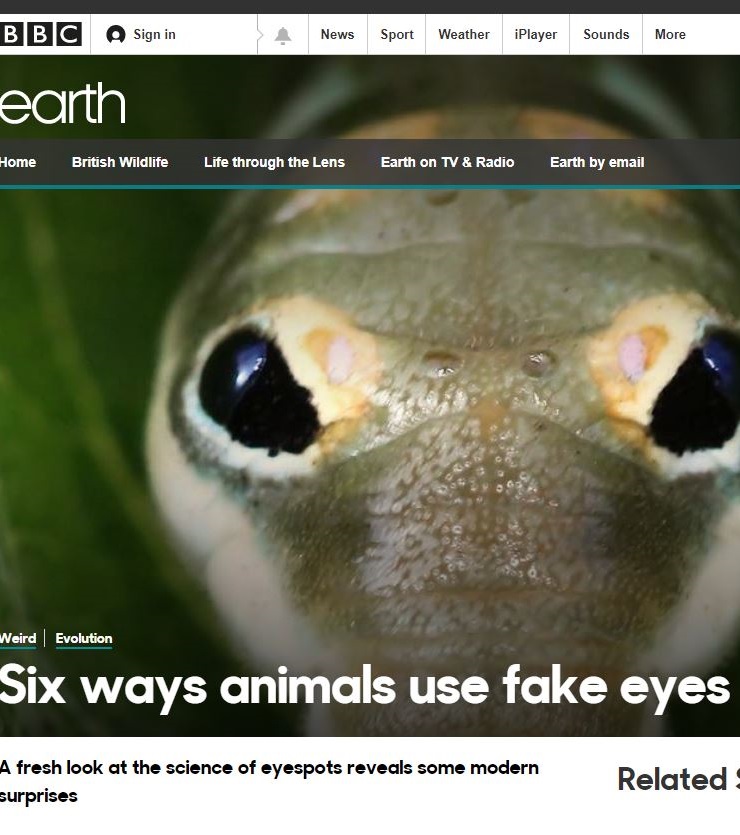A close-up image of a reptile's face, likely a turtle or lizard, with striking eyes and nostrils prominently featured. Patches of pink and cream are visible around its eyes, which are glossy and dark, adding to the creature's intense expression. Surrounding the creature are varying shades of green, highlighting the lush environment. The upper left corner of the image displays the BBC logo, followed by icons for signing in and notifications. The header includes options such as News, Sport, Weather, iPlayer, and Sounds. Below this is the Earth section, featuring links like Home, British Wildlife, Life Through the Lens, Earth on TV and Radio, and Earth by Email, separated by a thin green line. The headline below the photograph reads, "Weird and Evolution: Six Ways Animals Use Fake Eyes," introducing an article that explores the modern science behind eye spots, accompanied by an enticing glimpse of related content. The overall color palette of the image comprises white, black, yellow, green, brown, and subtle pink hues.